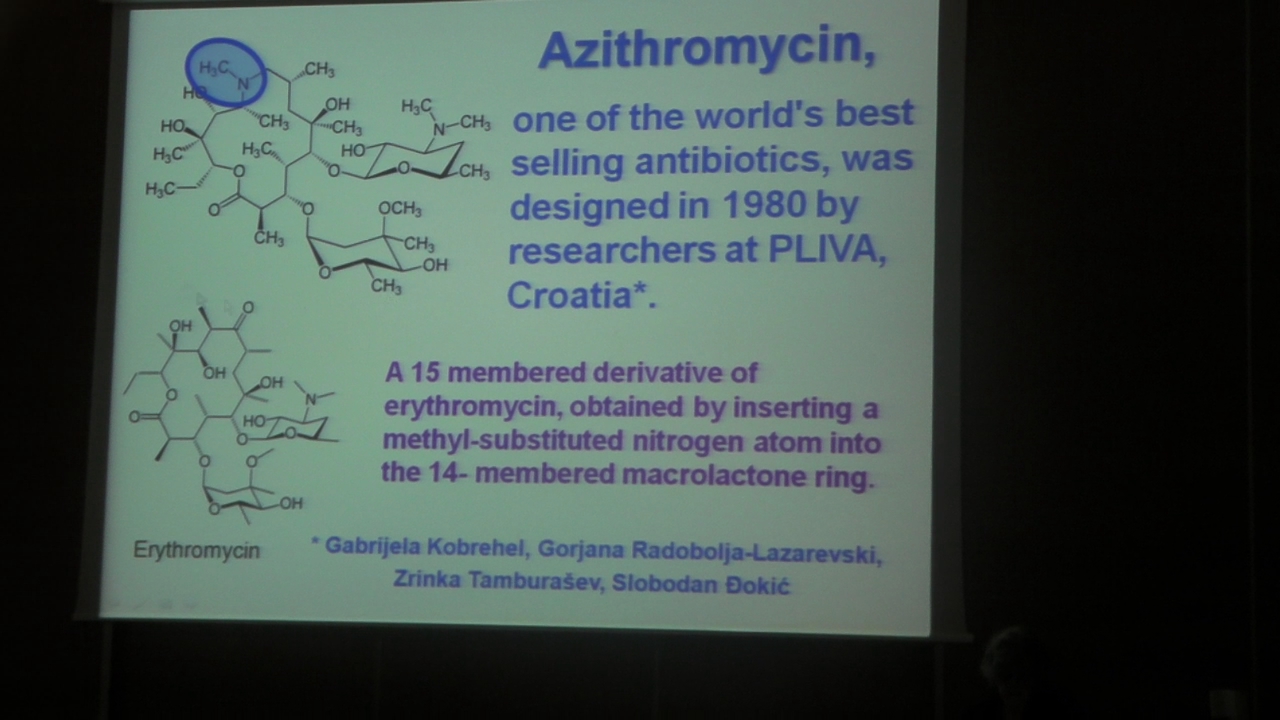The image appears to be a photograph of a scientific slide or poster, likely displayed on a screen or a piece of paper, with a white background and detailed scientific information about the antibiotic Azithromycin. The primary text is presented in blue and purple. At the top, it reads "Azithromycin," described as one of the world's best-selling antibiotics, designed in 1980 by researchers at Pliva, Croatia. Below this main title, in purple text, it explains that Azithromycin is a 15-member derivative of Erythromycin, created by inserting a methyl-substituted nitrogen atom into a 14-member macrolactone ring. On the left side of the text are scientific illustrations, showcasing the chemical structures and detailed composition of the antibiotic, with visual representations of DNA structures or atoms. At the bottom of the slide, additional text appears to include names of contributors or additional researchers, possibly in a foreign language, listing individuals such as Gabriela Korhel, Gorgona Rabidula, and others.